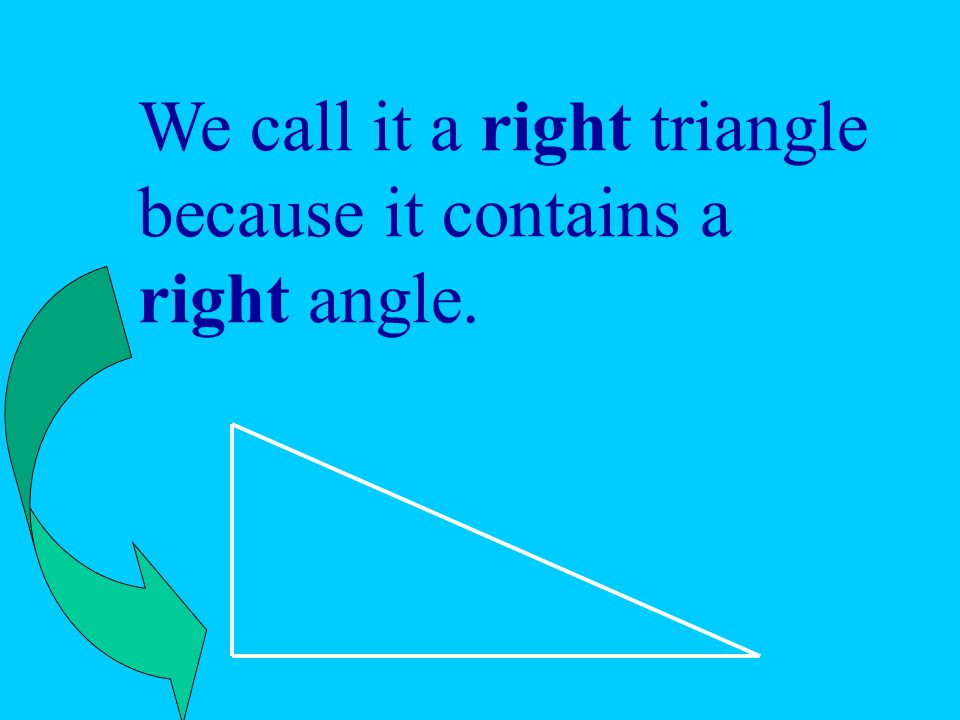This image, likely a slide from a mathematical presentation or an educational meme, features a baby blue, aqua-turquoise background. In bold, darker blue text at the top, it states, "We call it a right triangle because it contains a right angle." Emphasizing the key term, "right" is bolded both times it appears. Below the text, there is a white-outlined right-angled scalene triangle, seemingly tipped over with the longer side horizontal and the shorter side vertical. A distinctive, distorted green arrow, which transitions from a darker green at the top to a lighter green at the pointed end, swoops from the word "right" to the right angle within the triangle, clearly highlighting the triangle’s defining angle. The composition is simple and focused, with no other text or objects, making it a clear and effective visual aid for explaining the concept of right triangles.